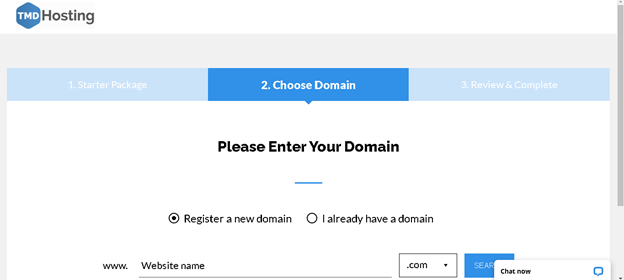This image is a screenshot of a website interface for a domain hosting service. In the top left corner, the website's logo features a blue hexagon with "TMD" in white letters inside it, followed by the word "Hosting" in black text.

The top banner of the website displays a three-step process for setting up hosting services. The first step, "Starter Package," and the third step, "Review and Complete," are represented in light blue rectangles with white text and are faded out, indicating that they are not the current steps. The second step, "Choose Domain," is highlighted in a bright blue rectangle with white text, signifying that this is the active step. A small downward-pointing triangle below this step further indicates that the user is currently on this page.

Centrally placed on the page, bold black text instructs the user to "Please enter your domain." Just below this instruction is a short blue line. Beneath this line, users are given two radio button options: "Register a new domain," which is selected with a black circle, and "I already have a domain." 

Following the radio buttons, there is a text input field prefixed by "www." where the user has entered "website name." Adjacent to this field is a dropdown box displaying the extension ".com." Next to the dropdown box appears a search bar, although only the partial text "SEAR" is visible because a "Chat Now" box is partially obscuring it. The chat box features black text reading "Chat Now" next to a blue message icon.